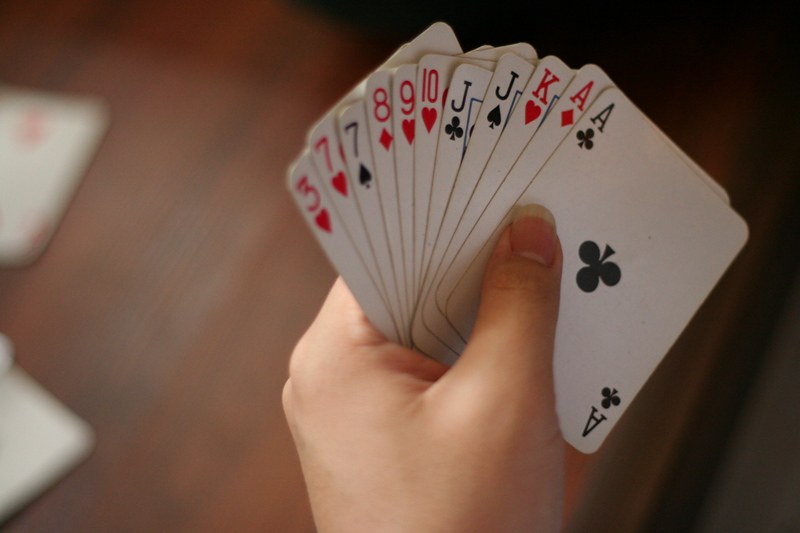In this image, a person is holding a spread of 11 playing cards in their hand. The background is a bit blurry but seems to feature a dark brown wooden table. On the left edge near the top, and positioned slightly downward, a card peeks out with a visible red mark, indicating it might be a heart or diamond. Below this, another card angles from the left down to the right and then sharply down to the left before disappearing from view; it's primarily white, with no visible markings.

At the bottom center of the image, the side of a hand is visible, with the thumb resting on top of the deck of cards. You can also see the area between the thumb and index finger, and the first two knuckles, while the fingers wrap around behind the cards. The cards are slightly fanned out, with the left side a bit closer to the camera, suggesting an effort to keep them from overlapping too much.

Starting from the left and moving clockwise, the visible cards are as follows: a 3 of hearts, 7 of hearts, 7 of spades, 8 of diamonds, 9 of hearts, 10 of hearts, Jack of clubs, Jack of spades, King of hearts, Ace of diamonds, and Ace of clubs. The thumb is placed particularly on the Ace of clubs, just to the left of the central club symbol on the card.